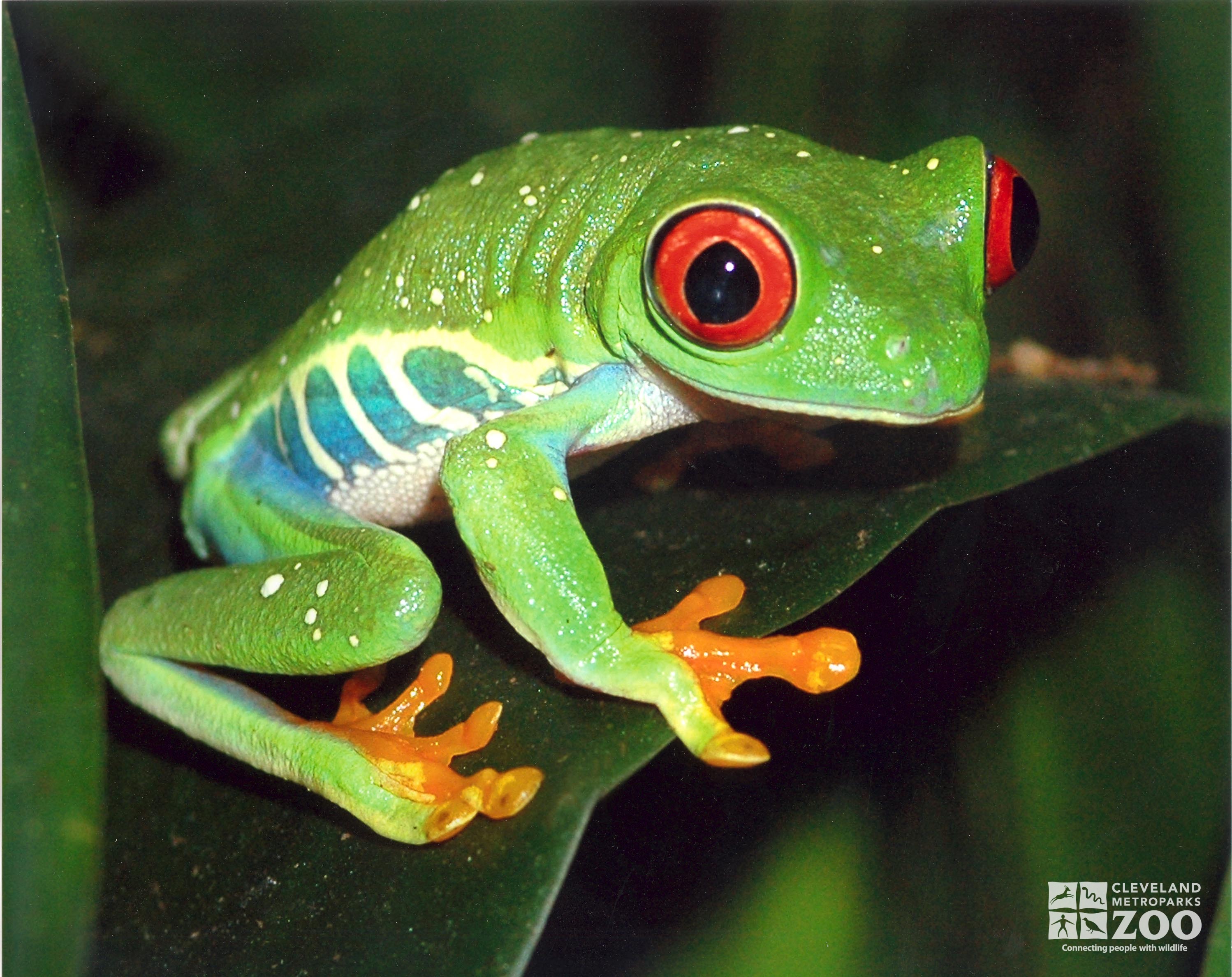This captivating photograph from the Cleveland Metroparks Zoo showcases an exquisitely colorful tropical rainforest frog perched on a broad, green leaf. The frog's vivid lime-green body is adorned with cream-colored speckles and exhibits a textured appearance reminiscent of a lime. Its large, bright red eyes, each with striking black pupils, are a focal point of its charming yet exotic look. The frog's underbelly features a white base with distinct blue stripes that extend partially up its sides, adding to its vibrant palette. A hint of blue is also visible at its arm joint with the shoulder. The frog's toes are a striking tangerine orange, adding to its overall flamboyance. Behind the frog, the background is softly blurred, highlighting the lush greenery and allowing the detailed beauty of the frog to take center stage. In the bottom right-hand corner, the logo of the Cleveland Metroparks Zoo appears, alongside silhouettes likely depicting a gazelle, a snake, a pheasant, and a gorilla, accompanied by the phrase "Connecting People with Wildlife." This image captures the essence of the zoo's mission to engage visitors with the wonders of the natural world.